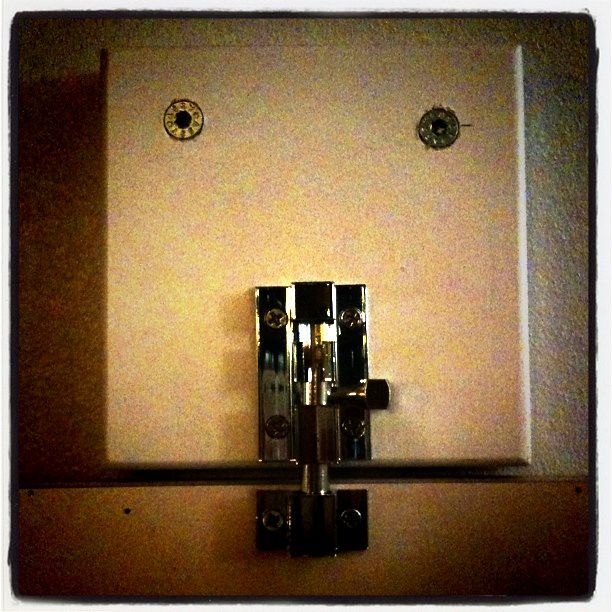This detailed photograph, presented in a square format with a thin white border, primarily features a door lock mechanism. The central subject is a chrome-colored, sliding bolt lock, typically seen on apartment and hotel doors. Positioned vertically in the center near the bottom of the image, the lock is in its secured state, with the deadbolt engaged in the latch.

The upper section of the image, covering about two-thirds of the frame, showcases a light tan wall. Centrally mounted on this wall is a raised square panel of a lighter tan hue, adorned with two circular, possibly star or hexagon-configured screws in its upper left and right corners.

Below the square panel, occupying the last fifth of the wall at the bottom, is a horizontal, raised rectangular area. This section serves as the mounting base for the lower part of the lock. The lock itself is fixed into place with four Phillips head screws on the square panel and two additional Phillips head screws secure the lower portion to the horizontal base.

The color scheme of the image is meticulously balanced, with the center appearing lighter compared to the outer corners, providing a subtle yet effective visual focus on the lock mechanism. The overall composition is a realistic, close-up portrayal of the lock against its background, capturing the fine details with photographic precision.